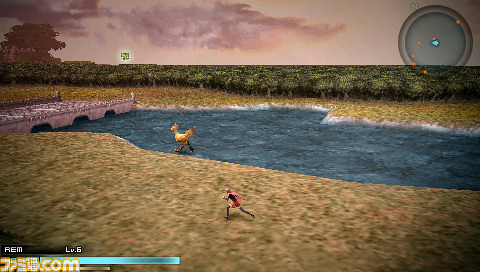A vividly detailed video game level is depicted in this image. In the bottom left corner, a multi-colored bar comprising mint green, light green, and blue shades is displayed, annotated with "REM level 6" and abbreviated as "LV6" just above it. Below the bar, yellow text reads "something.com." In the central viewing area, a brown ground base supports two characters: a small one, displayed in a side view, with pink and black coloring, and ahead of it, a yellow, chicken-like character running on what appears to be a blue ground base, possibly representing water. To the left of these characters, a gray bridge stretches above the scene, complemented by a series of green bushes and plants in the background. On the right side, a circular map icon features six orange dots along with a blue arrow. The sky overhead is a gradient of purple and pink hues, completing the enchanting visual.